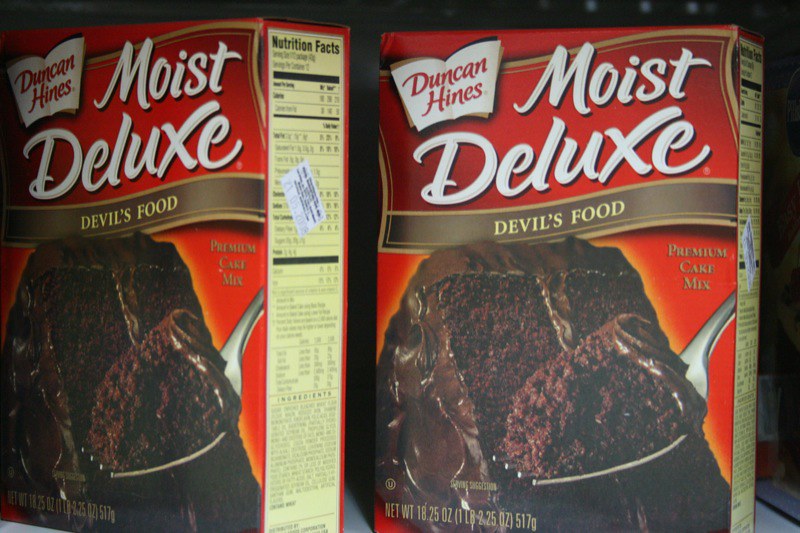The image features two boxes of Duncan Hines Moist Deluxe Premium Cake Mix, Devil's Food variety. Each box prominently displays vibrant red packaging with a large, enticing photograph of a rich, chocolate cake at the bottom center. A fork holds a moist section of the cake up towards the viewer, emphasizing its texture and appeal. The weight of the box, 18.25 ounces, is clearly indicated in elegant golden font at the bottom left corner. To the right side of each box, nutritional information is neatly presented on a beige background with black font. At the top left, the Duncan Hines logo is highlighted in red, set against what appears to be a stylized recipe book, with the words "Moist Deluxe" in crisp white font. Additionally, each box has pricing stickers or expiration dates affixed above the nutritional facts section on the right side.